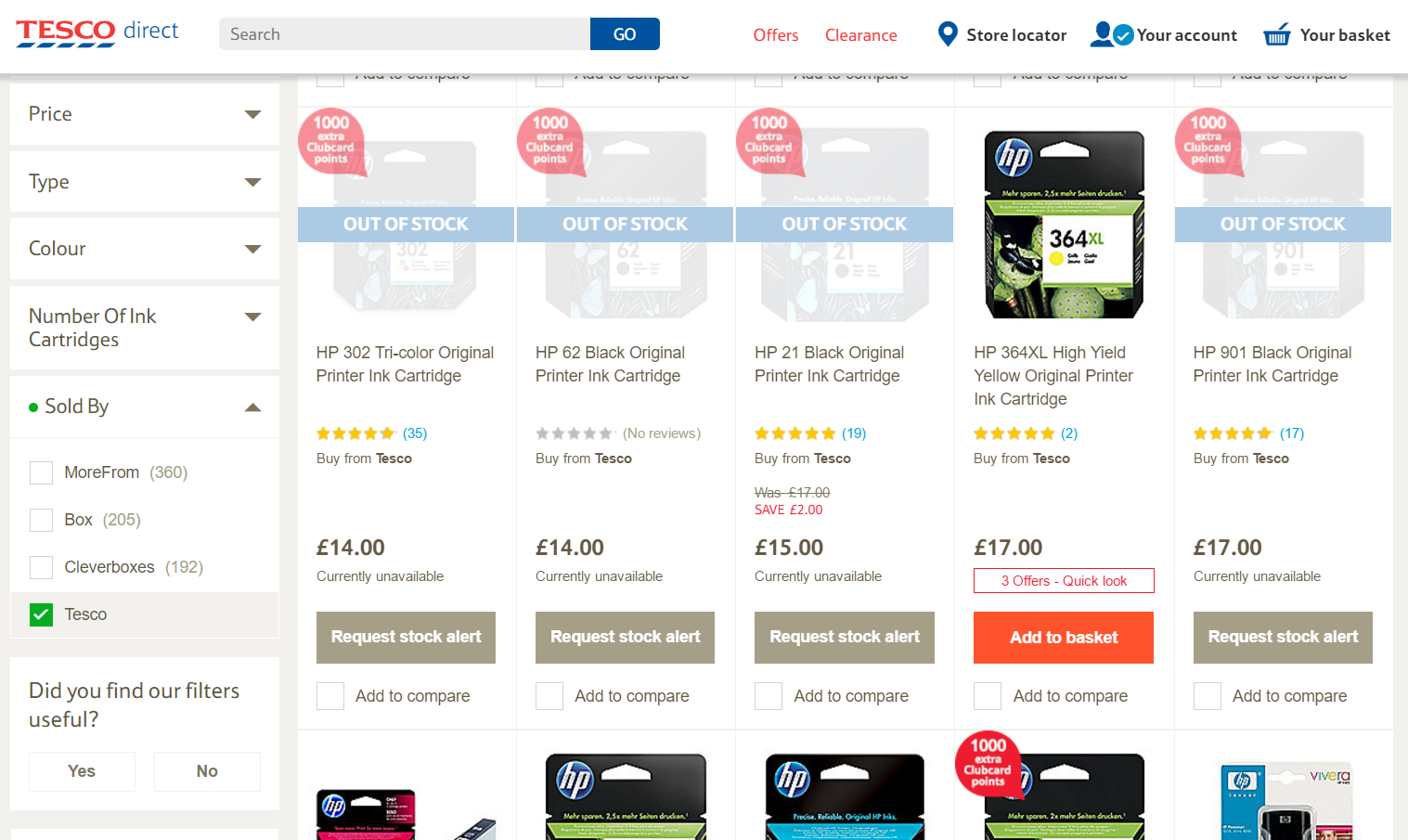This detailed screenshot from Tesco Direct's online store displays various features. At the top left corner, the Tesco logo is prominently shown with "Tesco" in red letters and "Direct" in blue letters. The site features a navigation bar with a search bar containing a "Go" button, alongside links to "Offers," "Clearance," "Store Locator," "Your Account," and "Your Basket."

On the left side, a vertical menu allows users to filter products by Price, Type, Color, Number of Ink Cartridges, Sold By, among other criteria. The filters include price points such as $3.60, $2.05, $1.92, and various vendors including "Clever Boxes" and "Tesco." Additionally, there is a customer feedback section asking "Did You Find Our Filters Useful?" with options for "Yes" and "No."

In the main area, several HP ink cartridges are listed. The "HP 302 Tri-Color Original Printer Ink Cartridge" is rated 5-stars, priced at £14, but it is currently unavailable, offering options to "Request Stock Alert" and "Add To Compare," with the promise of 1,000 extra Club Card points. Similar details are shown for the "HP 62 Black Original Printer Ink Cartridge" which has no reviews, and is also priced at £14 and unavailable.

The "HP 21 Black Original Printer Ink Cartridge" has a 5-star rating, was originally £17, now available for £15, but is also currently out of stock. The "HP 364 XL High Yield Yellow Original Printer Ink Cartridge" is highly rated at 5-stars, priced at £17 with 3 offers available, and includes options for "Quick Look," "Add To Basket," and "Add To Compare."

Lastly, the "HP 901 Black Original Printer Ink Cartridge," also with a 5-star rating, is priced at £17 and marked as currently unavailable with an option to "Request Stock Alert" and "Add To Compare." Each product listing highlights the offer of 1,000 extra Club Card points with purchase.